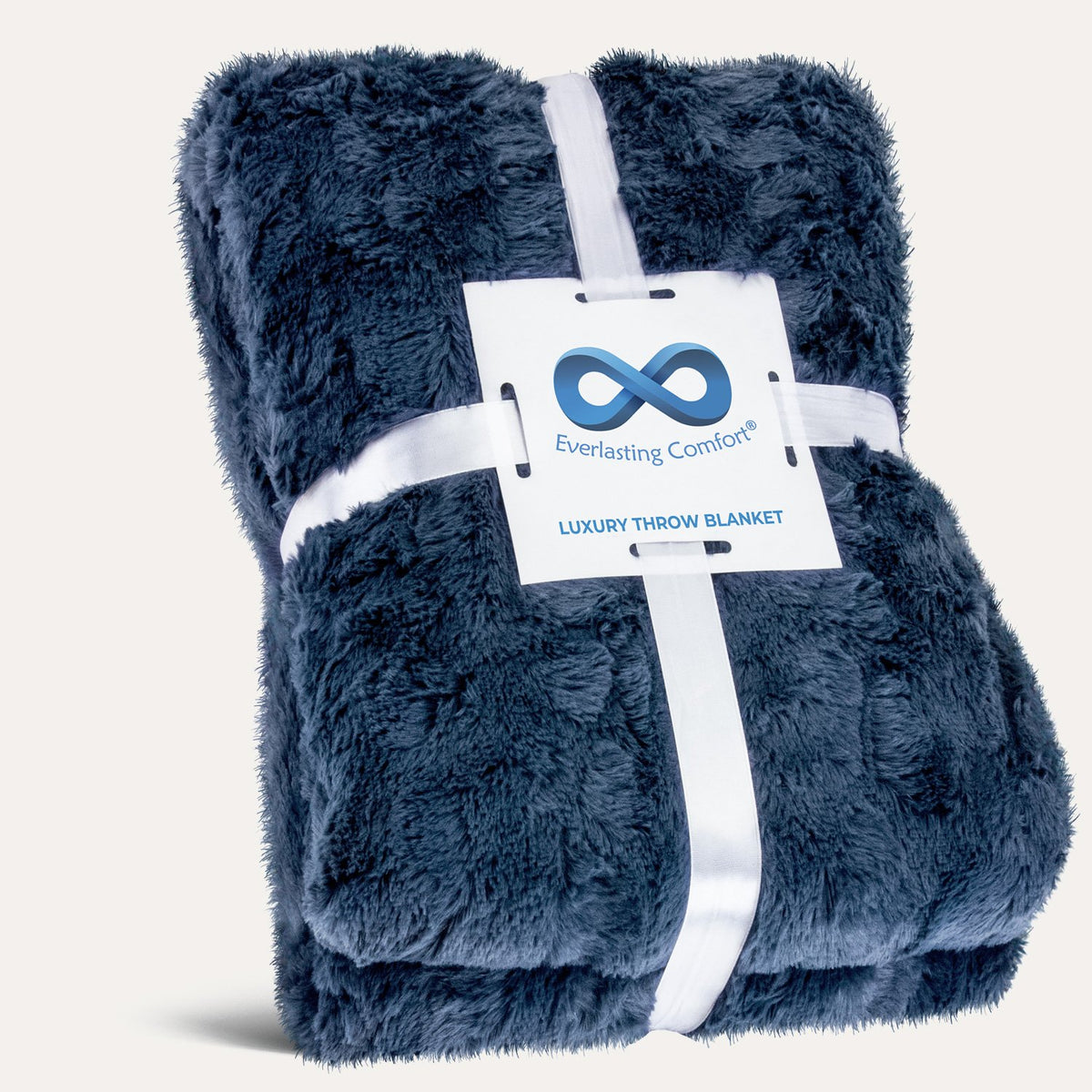This angled product image showcases a luxurious royal blue plush fur blanket, folded neatly in two, and presented against a white background. The blanket is secured with a white ribbon that criss-crosses around it, with some of the plush fur laying over the ribbon, adding to its cozy appearance. In the center of the blanket, there is a white square tag featuring the brand name "Everlasting Comfort" in blue letters, accompanied by a blue infinity symbol. Below the brand name, the tag states "Luxury Throw Blanket" in blue capital letters. The blanket appears to be propped up vertically, and its rich, dark blue color and fluffy texture give it an inviting, high-quality feel.